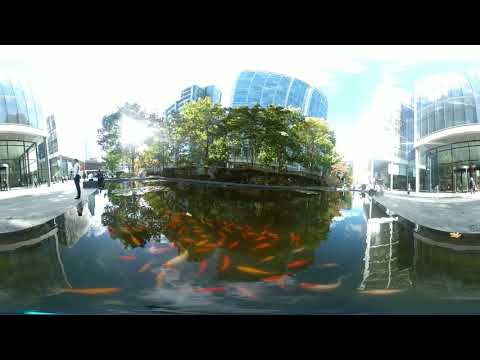The image captures a sunlit outdoor pond situated between several modern buildings with large glass windows. The pond, filled with around fifty large reddish-orange and light orange fish, has clear water that reveals dark undertones at the bottom. The concrete walkways on each side serve as paths for people to walk, with a few individuals visible in the frame. The buildings flanking the pond are two-story structures, characterized by glass facades and similar architectural features such as doors and awnings. Directly behind the pond, there's another glass-fronted building, lined with several trees in its front area. The photograph, taken with a GoPro, exhibits a slight distortion at the edges, giving the buildings an oval appearance and the scene a unique perspective. The entire scene is bathed in ample daylight, enhancing the overall brightness and clarity of the moment.